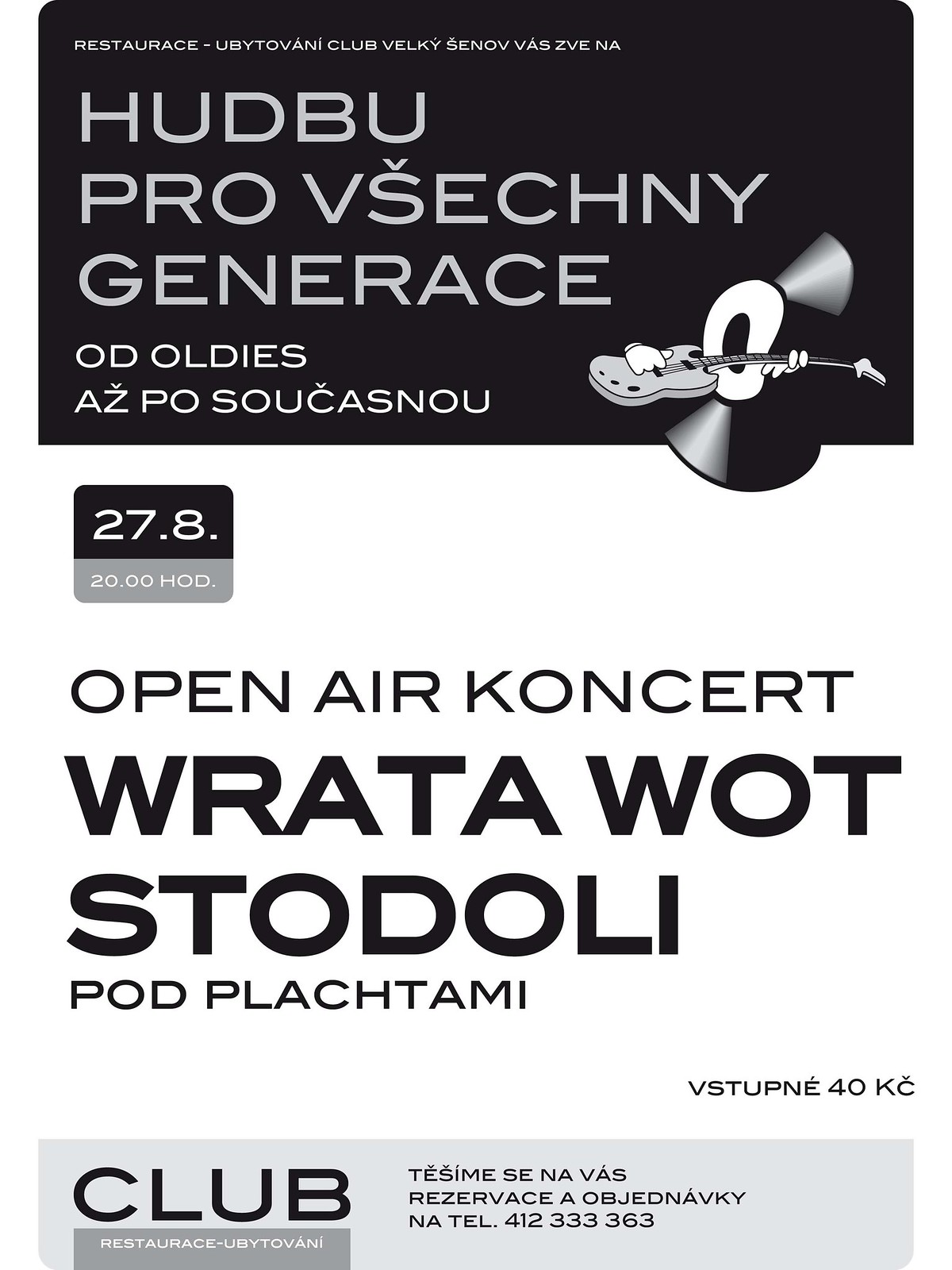This advertisement flyer for an open-air concert is predominantly black and white with bold, black typography set against a solid white background. The top section features a black rectangle with gray text, displaying a name or phrase that appears to be in German, beginning with "Hoodboo" and followed by words like "Pro Vazenshi Genarasi Odi Uldiz Azpo Sukhasnasu." Below that, the flyer announces the event as an "Open Air Concert," mentioning "Rata Wat Stadoli Pod Plaktami," presumably details related to the concert itself. Towards the bottom, the flyer clearly states "Club Restaurant," and includes a telephone number and address. Additionally, there is an illustration of a record holding and playing a guitar, emphasizing the musical nature of the event. Although the exact date is hard to decipher beyond a possible indication of 27.8, the flyer leaves no doubt that it is promoting a concert, even without a clear band name or concert type specified.